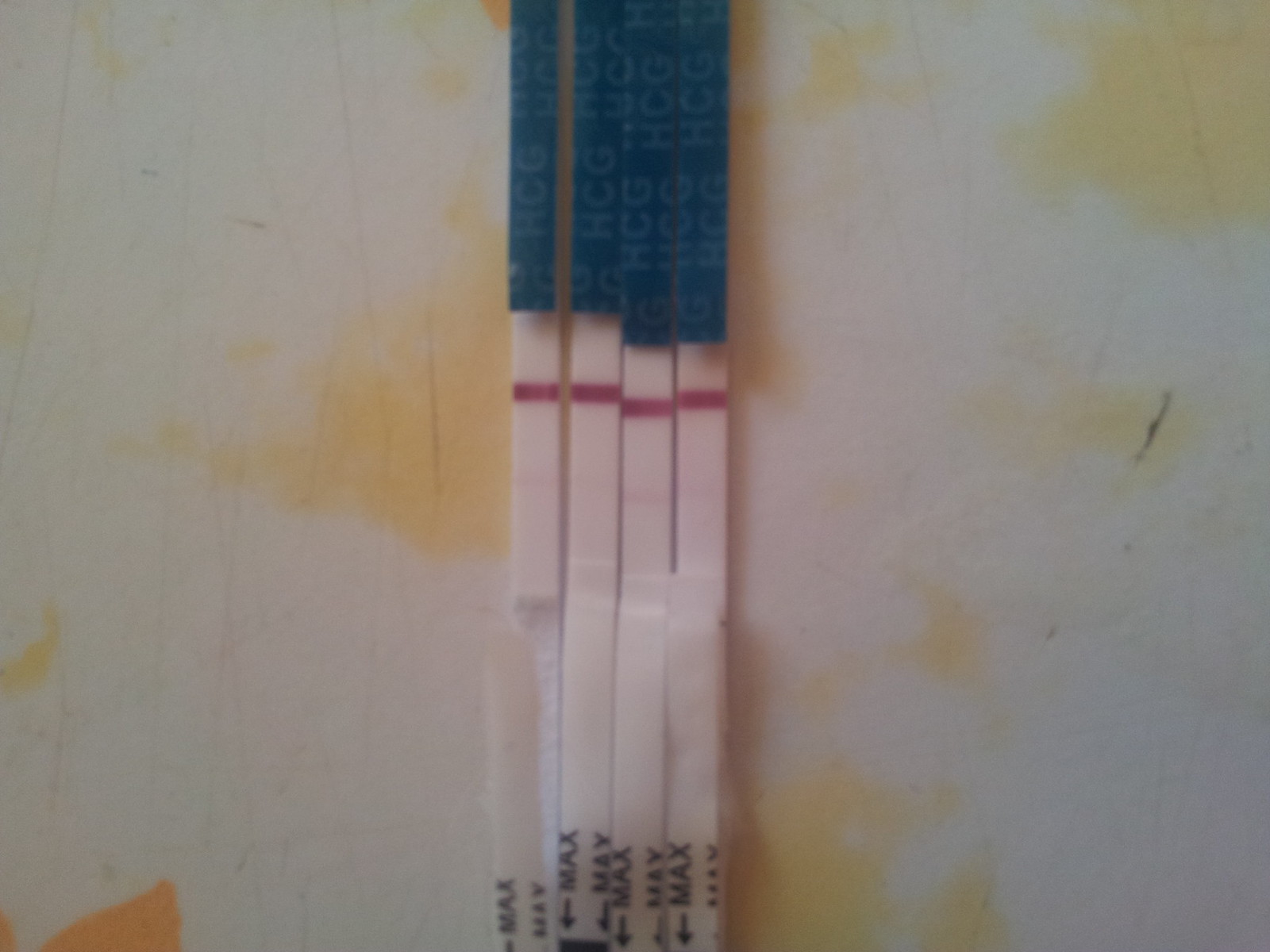The image features four white HCG test strips prominently centered on a somewhat stained and scraped white surface. Each strip displays a pink line running through the middle. At the top of the image, "HCG" is written in blue, accompanied by blue wrapping material. The bottom of the strips is marked with the word "MAX" and downward-pointing arrows. The white surface on which the strips rest is dotted with several yellow stains, predominantly located at the bottom, middle left, and top right sections of the image. Additionally, the bottom left corner of the surface showcases an orange stain, while smaller yellow blotches appear in the middle right and bottom left areas. A black speck of dust or debris is visible on the right side of the surface, and various scrapes and lines are scattered across it, contributing to a worn appearance.